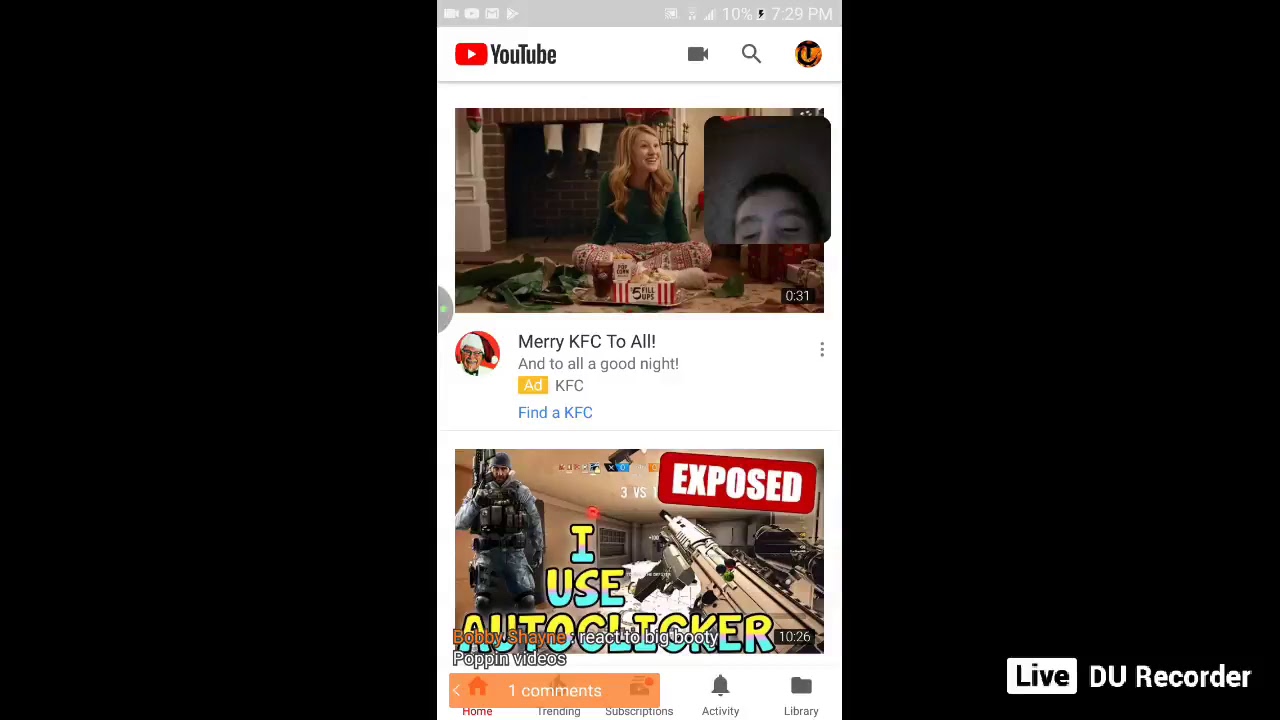The image is a landscape-oriented, color screenshot of a smartphone's screen, with notable black margins on both sides, making the actual displayed screen appear as a slim strip in the center. In the bottom right corner, there is a "LIVE" label from the DU Recorder app, indicating the screen is being recorded live.

Focusing on the details of the screenshot itself, the phone shows it's 7:29 PM and has a low battery at 10%. The reception is decent but not full, and several apps are running in the background, including Gmail and a video app. 

The central focus of the screen is the YouTube app, which is actively being browsed by the phone's user. The visible YouTube feed highlights two videos prominently. The first video, titled "Merry KFC to all," displays a young woman sitting on the floor, eating KFC, and conversing with someone off-screen. Below it, the second video is titled "I use auto clicker, exposed," showing a first-person shooter game image with a character in full military gear holding a gun.